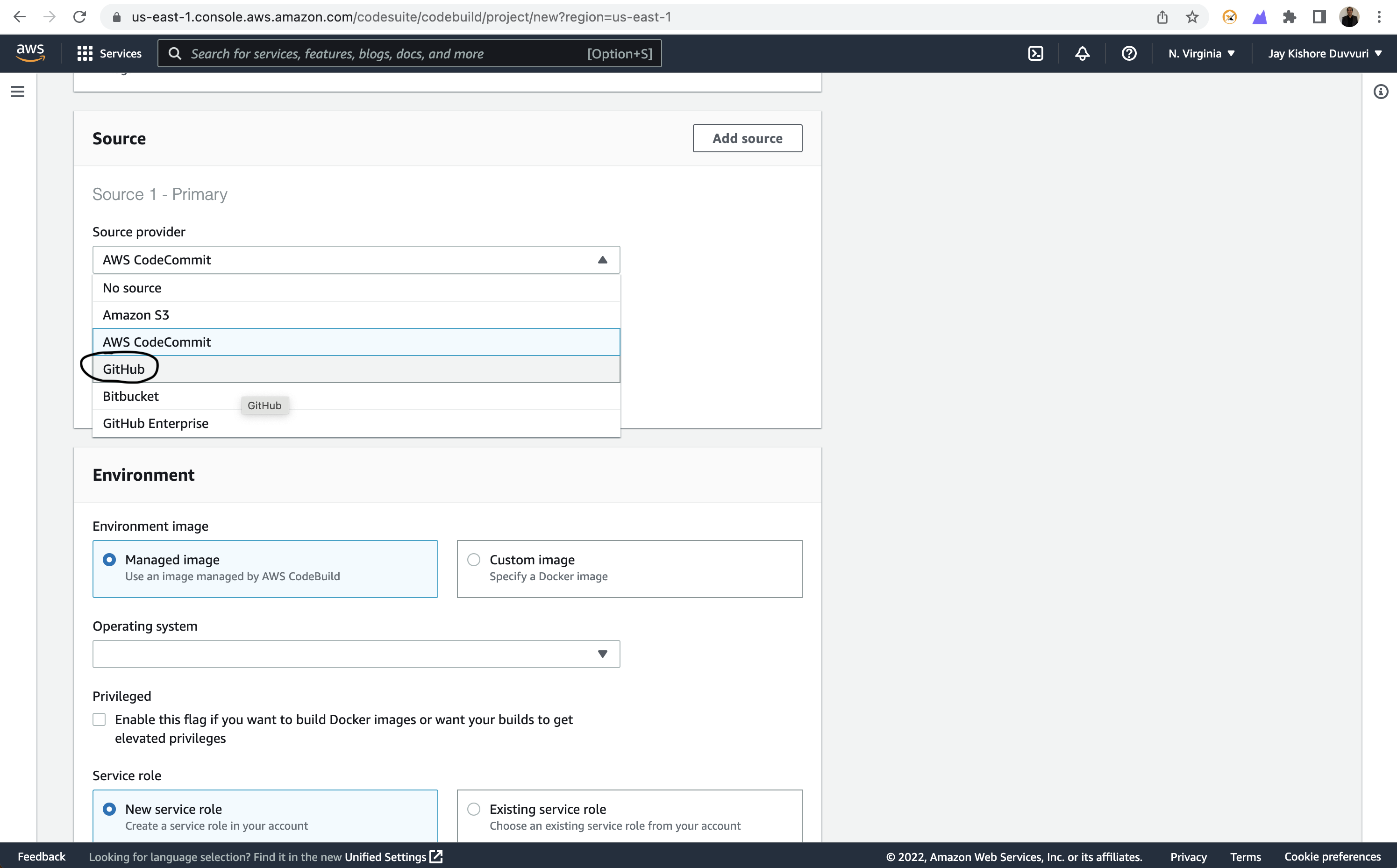**Caption: "AWS Configuration Interface - Detailed Overview"**

The image showcases an AWS (Amazon Web Services) configuration interface under the "Websites" category. At the top of the image, a black bar displays the AWS logo with "Services" and a search field labeled "Search for Services, Features, Blogs, Docs, and more."

Beneath the black bar, a gray background hosts multiple white boxes with various settings. The first white box, titled "Source," lists options such as "Source 1," "Primary," and "Source Provider." Below these are selections for "AWS Code Commit" and other providers like "GitHub" (which is circled), "Bitbucket," and "GitHub Enterprise."

The next box is labeled "Environment." It provides options for "Environment Image," with choices including "Manual Image" and "Custom Image," as well as an "Operating System" drop-down menu.

Further down, a section on "Privileges" includes an option to enable elevated privileges for building Docker images.

Lastly, the "Service Role" section allows users to either create a new service role by checking "New Service Role" or select an existing role by choosing "Existing Service Role."